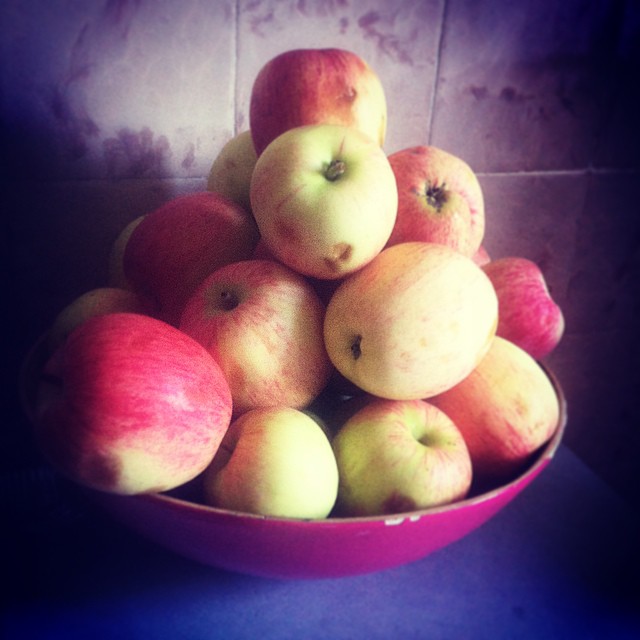The image depicts a chipped red bowl stacked high with a mixture of red, yellow, and green apples, many of which have noticeable brown spots and dents, indicating they are overripe or starting to rot. The bowl, chipped around the edges to reveal white beneath, holds approximately 18 to 20 apples arranged in a pyramid-like fashion, and is set on a blue countertop. The backdrop features a tiled wall with hues varying from grayish-white to light purple, adding to the overall muted and somewhat dark ambiance of the scene.